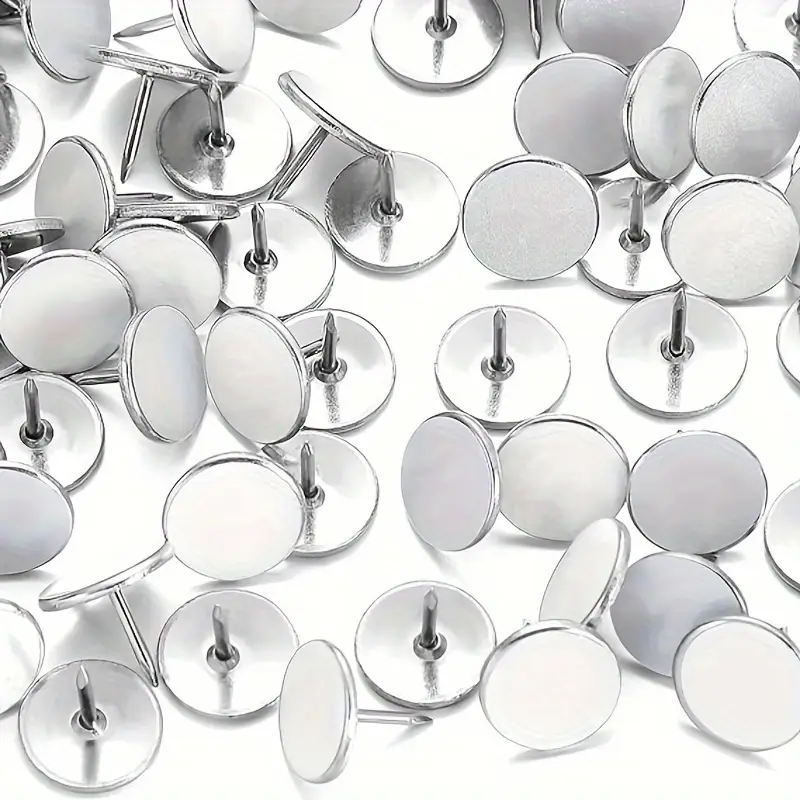The image showcases a large collection of approximately 30 to 40 tacks set against a crisp white background. These tacks feature a glossy white, circular top with a silver underside and a sharp, silver needle point. Their arrangement appears random, with some tacks lying on their backs, thus displaying only the circular tops, while others rest on their sides, revealing both the pointy needles and the tops. The tacks are sporadically scattered across the image, creating clusters in some areas where the background is barely visible, whereas in other areas, the white backdrop is more prominent. The overall scene is a zoomed-in perspective of these tacks casually strewn across a flat surface.